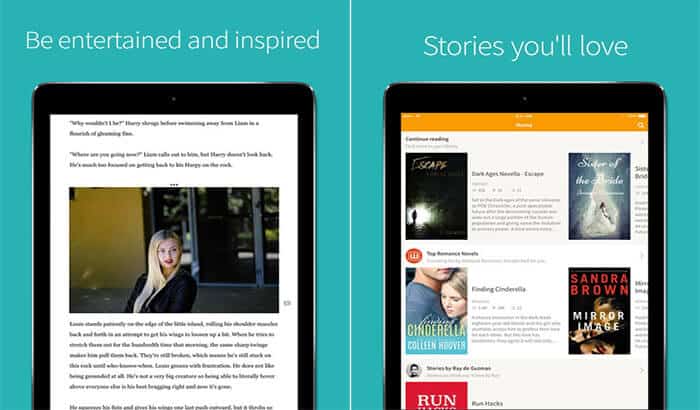The advertisement features a wide, turquoise background with white text at the top. A white line splits the image down the middle, with a picture of a tablet on each side.

On the left side, the tablet displays what appears to be an article. The screen shows a significant amount of black text on a white background, interspersed with a large image of a young, blonde woman with bright red lipstick, photographed from the torso up in front of glass doors. Above the image, white text reads, "Be Entertained and Inspired," while beside it, more white text says, "Stories You'll Love."

On the right side, the tablet screen showcases a book-reading app, displaying the covers of five different books. The text on the screen reads, "Continue Reading," and among the visible book covers are titles such as "Mirror Image" by Sandra Brown, "Finding Cinderella" by Colleen Hoover, and "Sister of the Bride."

The clean and vibrant design, featuring both article content and book recommendations, aims to entice viewers with a blend of entertainment and reading inspiration.